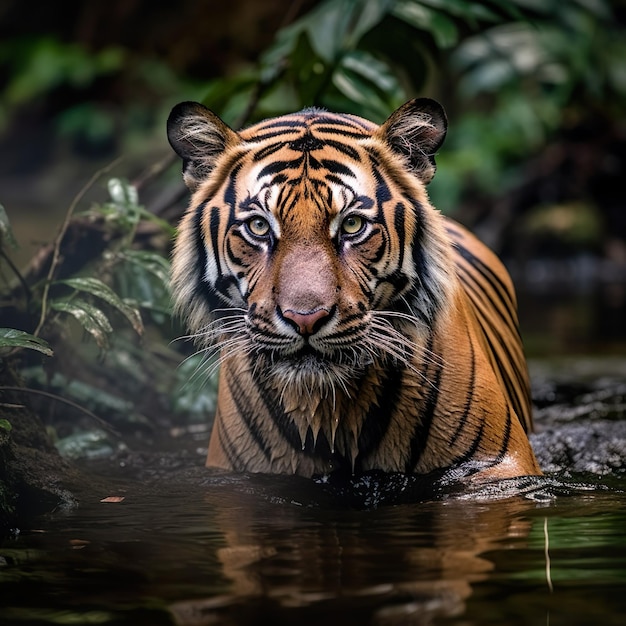The image depicts a close-up of a tiger standing in a still body of water, reaching chest height, with water droplets visible under its chin. The tiger, showcasing the characteristic orange fur with black stripes and white accents on its face and neck, stares directly at the camera with light-colored eyes, which appear hazel green or light brown. Its fur looks wet and matted, particularly around the neck and upper chest. The tiger's pink snout and distinct whiskers are clearly visible, along with its furry, raised ears and an orange mane-like collar around its neck. In the background, some green leaves and brown branches from a fallen tree partially obscure the scene, adding a sense of depth and natural surroundings. The reflections of both the tiger and the foliage can be seen in the water, which remains mostly undisturbed, suggesting that the tiger might be moving slowly towards the camera. The setting appears shaded and tranquil, with a blurred glimpse of the ground in the far back left corner.